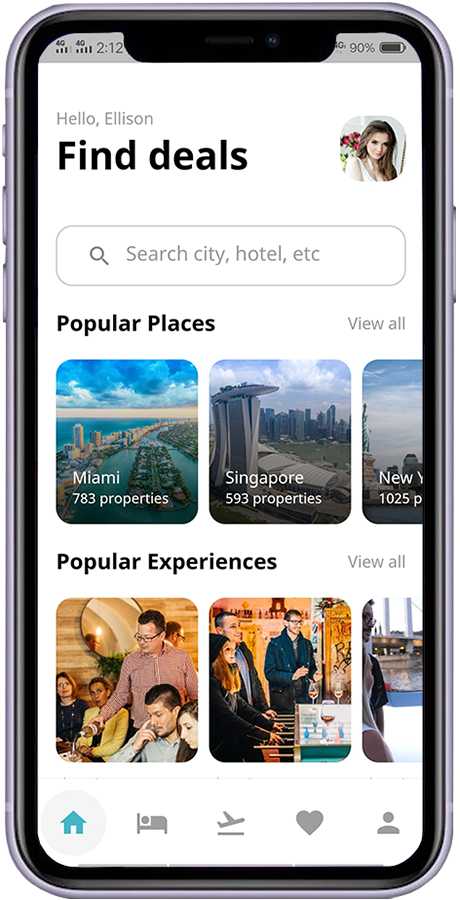In this image of a cell phone screen, the phone itself features a sleek, silver outline. On the left side of the device, there are three buttons, while a thicker button is visible on the right side. A black outline encircles the screen, followed by a grey segment at the top and another thicker black outline on the inner edge, creating an oval framing effect towards the upper portion of the display. The left and right edges of the screen display a slight grey tint.

At the top left corner, the font appears small but readable, indicating "212" in grey. The top right corner shows a battery status of "90%". Beneath this top section, the screen has a white background with greyish text that reads "Hello Ellison" on the left. Below this greeting, in black text, is the phrase "Fine Deals," accompanied by a picture of a Caucasian woman with dirty blonde hair wearing a white top. Red roses or flowers are noticeable behind her.

Further down, there's a grey-outlined circle with a magnifying glass icon in grey, marked by the text "Search City, Hotel, etc." Below this search bar, in black text, the screen displays "Popular Places." Three locations are listed: the first is Miami with 783 properties, showcased in a rounded box featuring a photograph of downtown Miami with a blue sky. The middle listing is Singapore with 593 properties, accompanied by a cityscape outline of Singapore. The third listing shows New York, displaying 1025 properties, though this image is partially cut off. Next to the "Popular Places" title, on the right, is the option "View All."

Further down, labeled "Popular Experiences" in black text with "View All" in grey to the right, three photographs are present: one depicting a waiter pouring wine in a restaurant, another showing people standing around a foosball table, and a third partially obscured image.

At the bottom of the screen, there are a series of icons: a blue house, a grey circle, a grey outline of a person laying in a bed, a plane taking off from flatland, a grey heart, and an image of someone's head and shoulders on the far right.